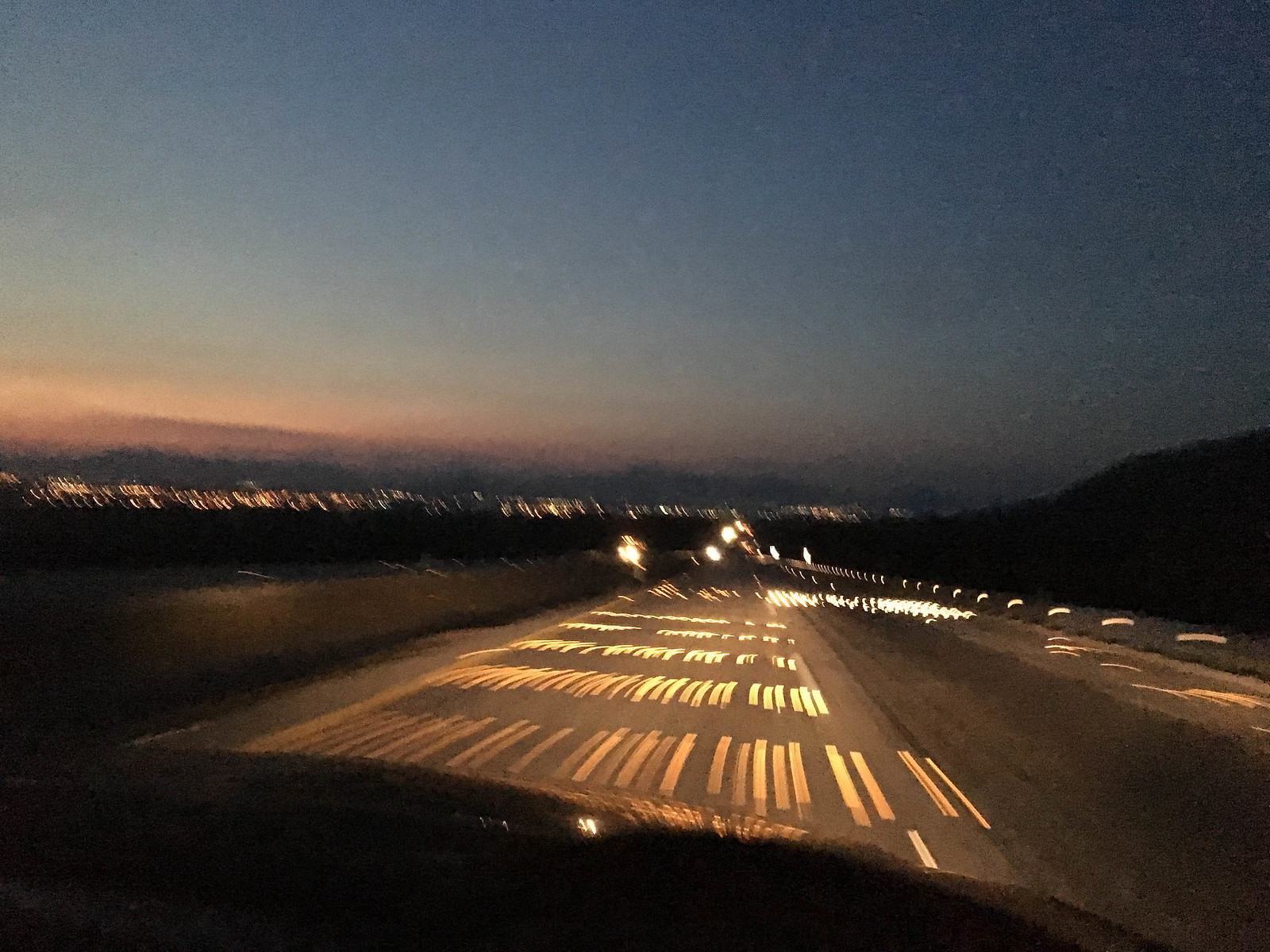This color photograph captures a dynamic night scene as viewed from inside a moving car. The sky above transitions from dark gray at the top to a blend of blue, pink, and light purple near the horizon, suggesting the sun has recently set. In the foreground, the road is illuminated by yellow lights, their glow enhanced by the motion blur. Four distinct vertical lines run along the street, leading to bright yellow sparks that appear to float and shimmer in the air. The right side of the road features a dark hill, while the left side is bordered by a gray wall. In the distance, a cityscape of blurred lights and buildings is visible against the darkening sky. The image, slightly blurry, emphasizes the movement and vibrant lighting of the scene, capturing the contrast between the illuminated road and the encroaching night.